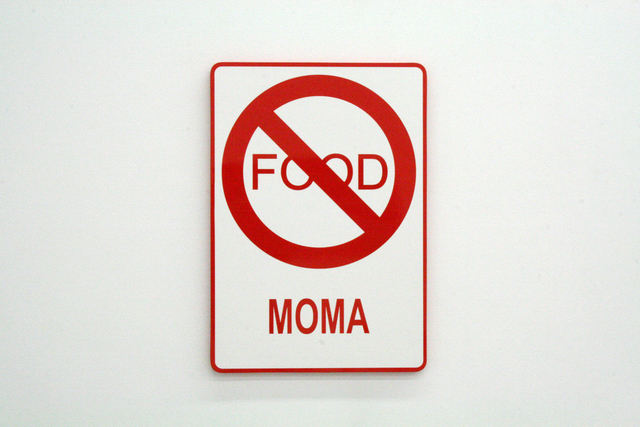The image features a vertically oriented, rectangular sign with rounded edges, centered against a light gray background. The sign has a thin red border and a white interior. Dominating the top two-thirds of the sign is a red circle with a diagonal line running from the upper left to the bottom right, crossing out the word "FOOD" written in thin, red, capital letters. Below this "no food" symbol, the word "MOMA" appears in the same red, capital letters. The overall composition is simple and minimalistic, focusing on the clear message conveyed by the sign's text and symbols against the neutral backdrop.